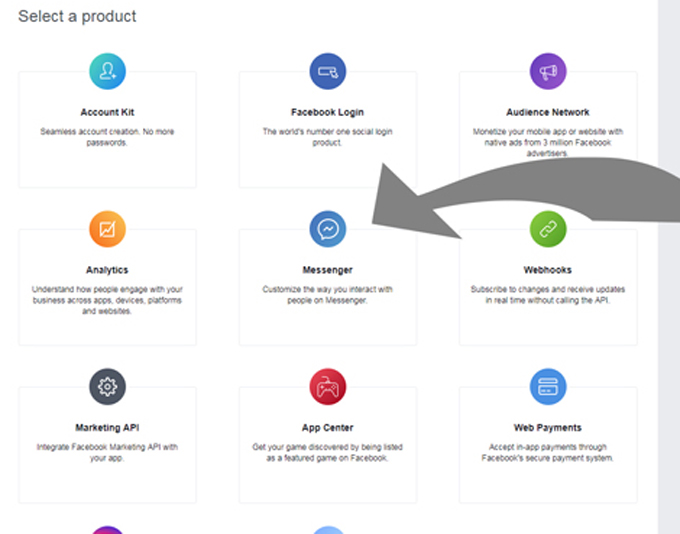The image depicts a 3x3 grid of square tiles, each containing a distinct circular icon. These icons vary depending on the application or service they represent. Some of the icons and their corresponding titles include:

- **Account Kit**: Facilitates seamless account creation, eliminating the need for passwords. Its tile is light blue.
- **Facebook Login**: Touted as the world's number one social login product, the icon is predominantly blue.
- **Audience Network**: Unknown icon description, but the tile is likely different in color.
- **Analytics**: Features an orange tile with a white graph-like icon.
- **Messenger**: Displays the Facebook Messenger icon on a light blue background.
- **Webhooks**: Icon and color are unspecified.
- **Marketing API**: Icon and color are unspecified.
- **App Center**: Contains a gaming controller icon set against a red background.
- **Web Payments**: Icon and color are unspecified.

Majority of the icons have a blue hue, although there are variations such as dark blue, purple, green, gray, red, and orange. There are more grids beyond the visible screen area.